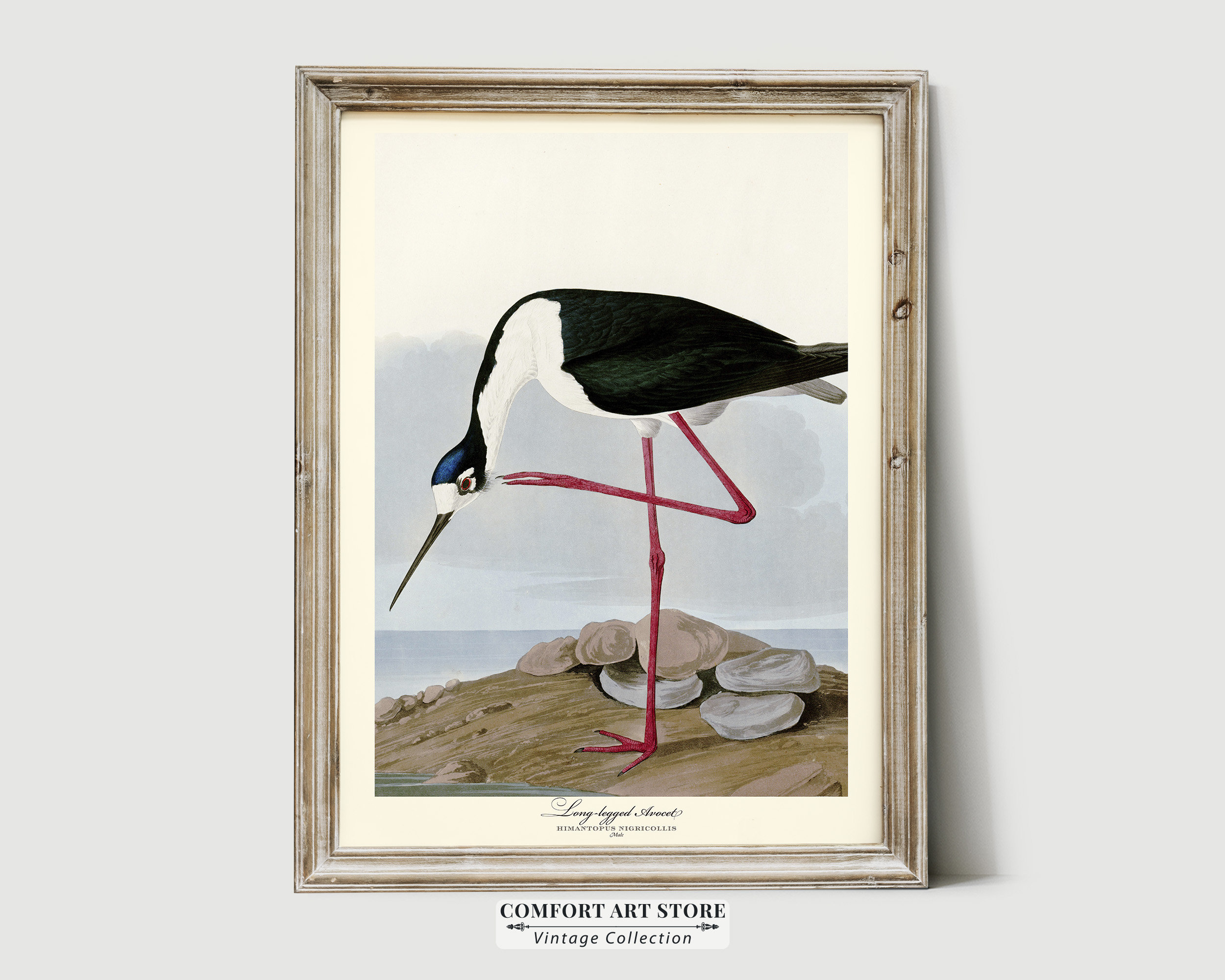This detailed photograph captures a vintage artwork from the Comfort Art Store's collection, elegantly framed in a light-colored wooden frame with a cream-colored border. The centerpiece of this artwork is a meticulously painted long-legged shorebird, likely a crane or heron, depicted with a striking combination of colors. The bird features reddish-pink legs, a black and white body, and a blue-toned forehead, along with a distinctive long black beak. The scene portrays the bird standing on one leg with the other bent toward its head, poised as if it's about to snatch something from the ground. The background reveals a natural coastal setting, with the bird perched near rocks, surrounded by sandy or grassy terrain, and with the ocean and a cloudy blue sky visible in the distance. An inscription below the painting marks it as part of the Comfort Art Store's well-maintained vintage collection, adding to the historic and artistic value of this captivating piece.